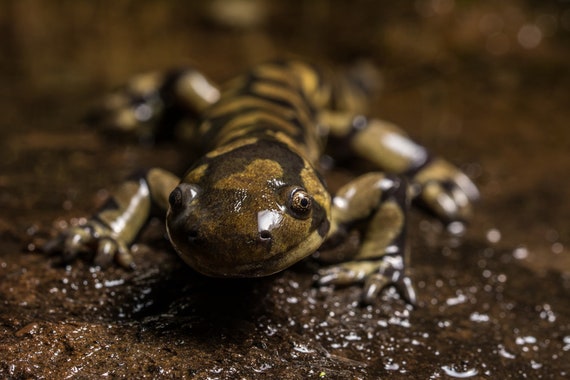The image features a vibrant, green amphibian-like creature with bug-like eyes and a nose with two holes, staring intently at the camera. It has distinctive yellow and black stripes running down its back, giving it a striking appearance. The creature's limbs are sharp and resemble those of a lizard, and its body appears to be slippery and slimy, hinting at its amphibious nature. The scene is set on a wet, muddy surface mixed with stone, reflecting the light and emphasizing the damp environment. This high-definition, nighttime photograph, likely taken by a wildlife photographer, captures not only the detailed markings of the frog-like animal but also the playful, almost animated quality of its form. The background is slightly blurred, maintaining the focus on the amphibian amidst its naturally wet surroundings.